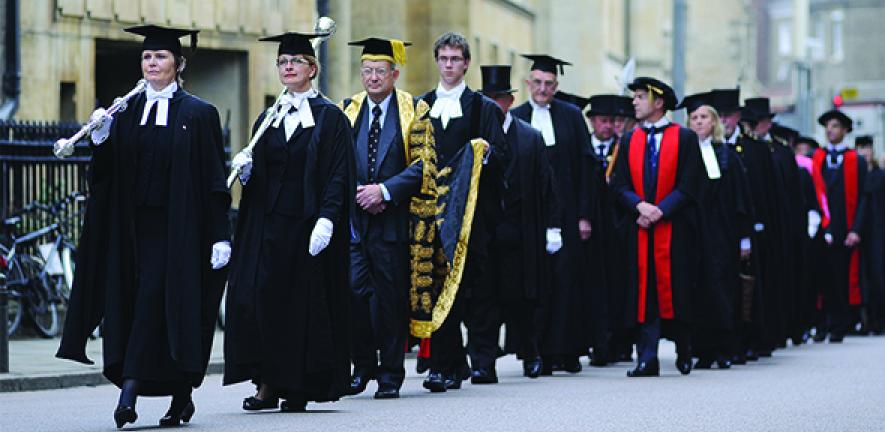In this horizontal rectangular image, a parade of graduates and scholars is progressing down a city street lined with buildings. They are all donned in black cap and gown ensembles, typical of graduation attire. The majority of them are also sporting white scarves, while some have an additional long red scarf draped around their robes. At the front of the procession, two older individuals are holding silver scepters and wearing pumps, standing out in their distinctive formal graduation caps. Among the noteworthy figures, one older person has a unique item draped around their shoulders, and right behind this individual, a younger person is carrying a large, antique gold-colored musical instrument. Another figure near the front is distinguished by a heavy yellow coat with blue accents and tassels on their hat, adding a splash of color to the otherwise monochromatic procession. The participants appear to vary in age, predominantly older individuals with a few younger ones interspersed, all moving in a mostly orderly line down the right side of the road, capturing a ceremonial and scholarly ambiance against the urban backdrop.